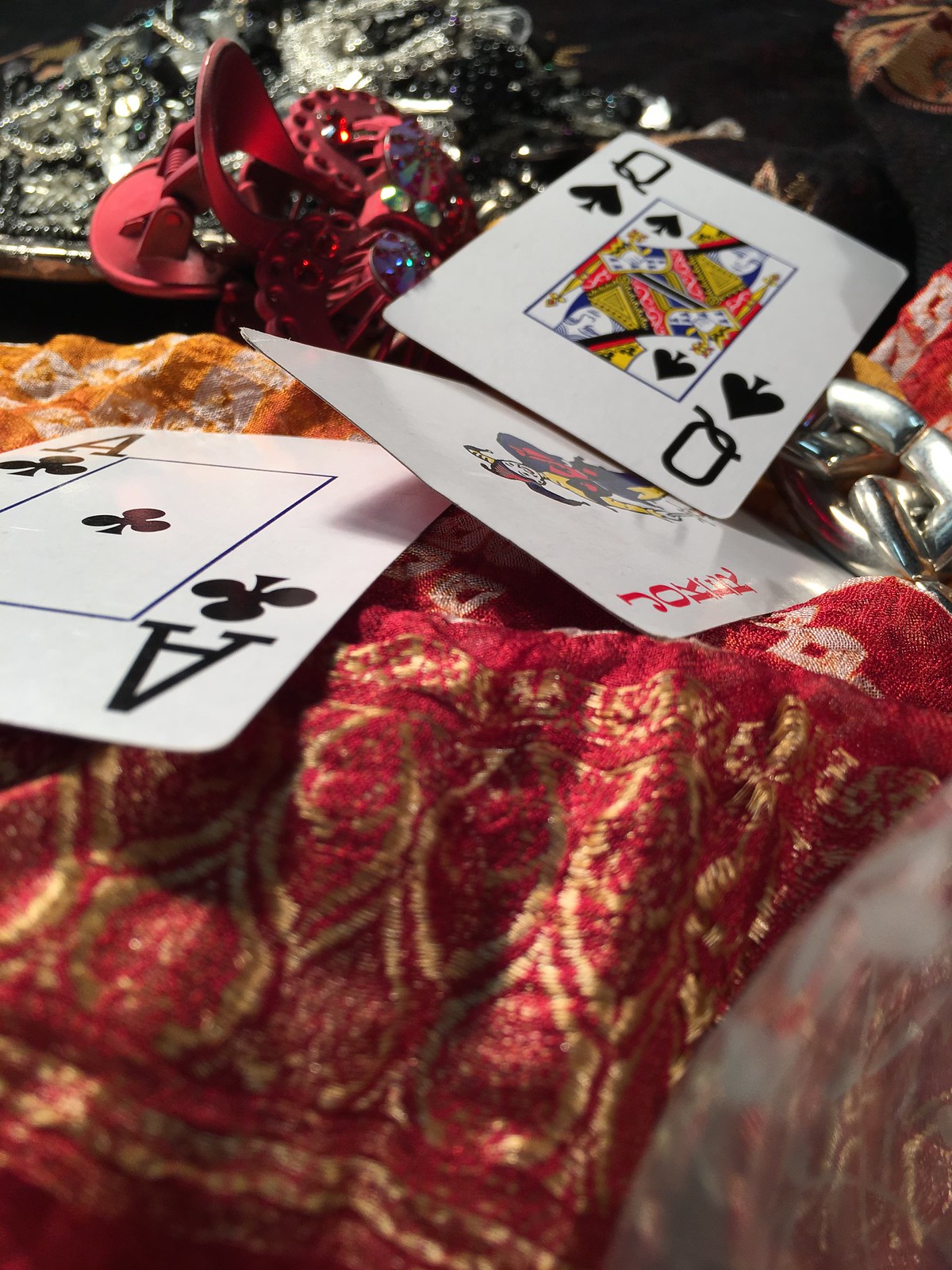In the image, three playing cards are carefully arranged atop a variety of silky fabrics. From left to right, the cards featured are the Ace of Clubs, a red Joker, and the Queen of Spades. The Ace of Clubs card is positioned such that its corner touches the back of the red Joker card. The red Joker card's front, in turn, meets the corner of the Queen of Spades card. 

The brightly colored silk fabrics underneath the cards add vibrancy to the scene. The fabric directly beneath the cards is a rich red adorned with yellow patterns. To the rear of this centerpiece, there are additional silks in shades of orange, another bright red, and a lustrous grey. The lighting in the image casts realistic shadows where the cards overlap, further enhancing the lifelike quality of the scene.